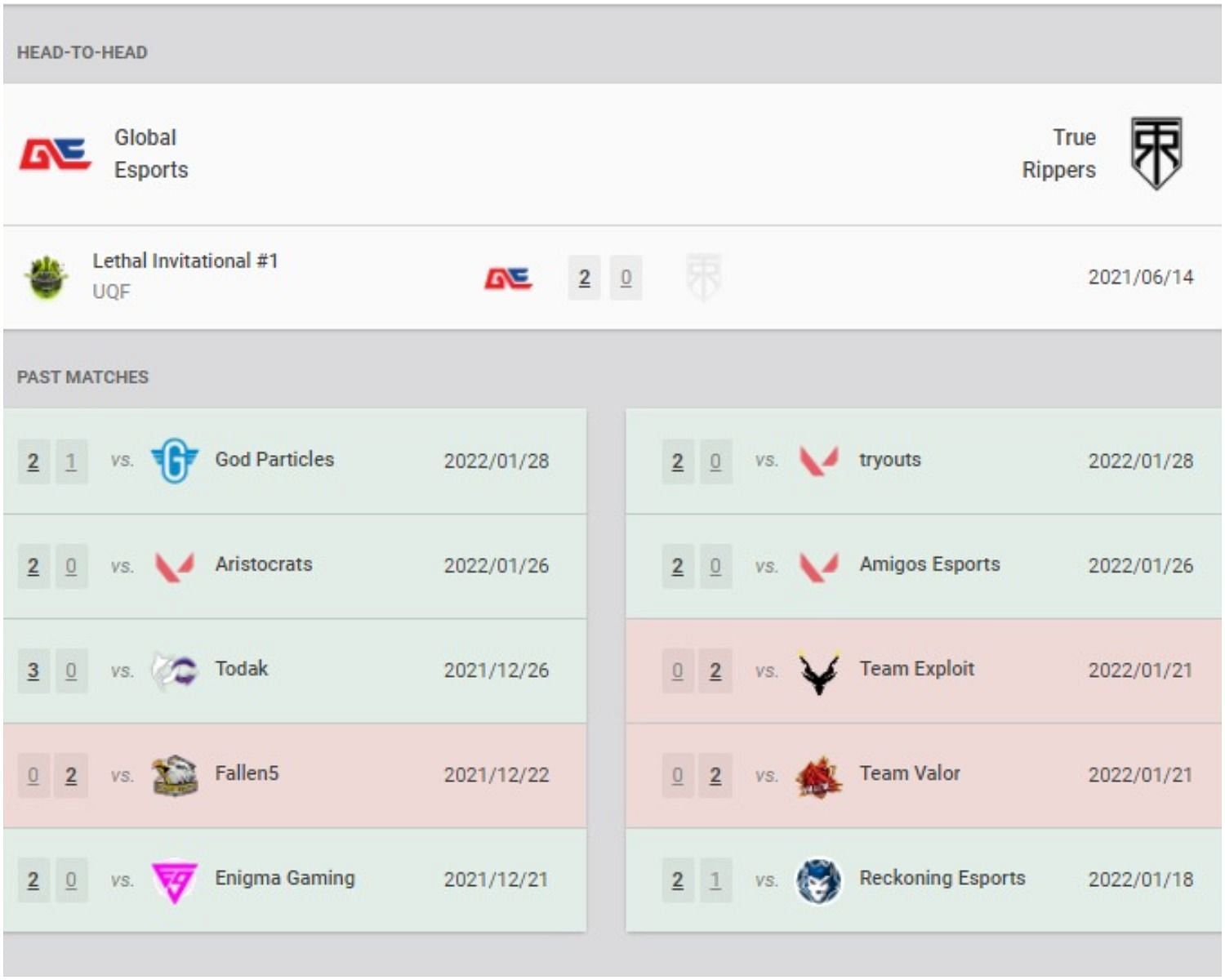This detailed caption provides an extensive description of a website screenshot, emphasizing the layout and elements contained within the captured image:

---

The screenshot captures a website displayed on a desktop or widescreen device, characterized by a light gray background and various sectional divisions with distinct background colors including white and light green. At the top of the screen, the heading "HEAD TO HEAD" is prominently displayed in all caps against a dark or light gray backdrop, featuring darker gray text.

Beneath the heading, a smaller section with a white background and a thin light gray dividing line runs horizontally across the screen. On the left side of this division, there is a red and blue logo adjacent to the text "Global Esports." On the right, the text "True Rippers" is paired with a black and white logo positioned to its right.

Below this, a further detail includes smaller text accompanied by a light green logo on the left that reads "LETHAL INVITATIONAL #1 UKF" in light gray text. On the right side of this division, beneath the thin dividing line, the date "2021-06-14" is displayed.

The section following this date features a list of past matches organized into two separate columns. Wins are highlighted in light green, while losses are marked in light red, providing a clear visual distinction between the outcomes of each listed match.

---

This caption gives a comprehensive and structured description of the website's layout, emphasizing each section's design and content elements.